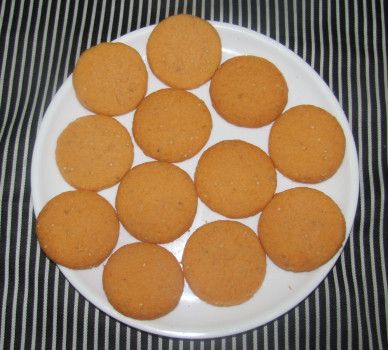A close-up image features a white dinner plate positioned at the center of a table adorned with a vertically striped black and white tablecloth. On the plate rests a dozen round cookies, each resembling a vanilla wafer in both shape and light brown color. These cookies are perfectly round and uniform in size, arranged in a neat, artsy pattern where they touch each other but do not stack. Their precise arrangement forms subtle triangular shapes between them. The photo, likely taken indoors, captures some crumbs scattered on the plate, hinting that the cookies have recently been handled. Light reflects softly off the plate, enhancing the intimate, homey feel of the setting.